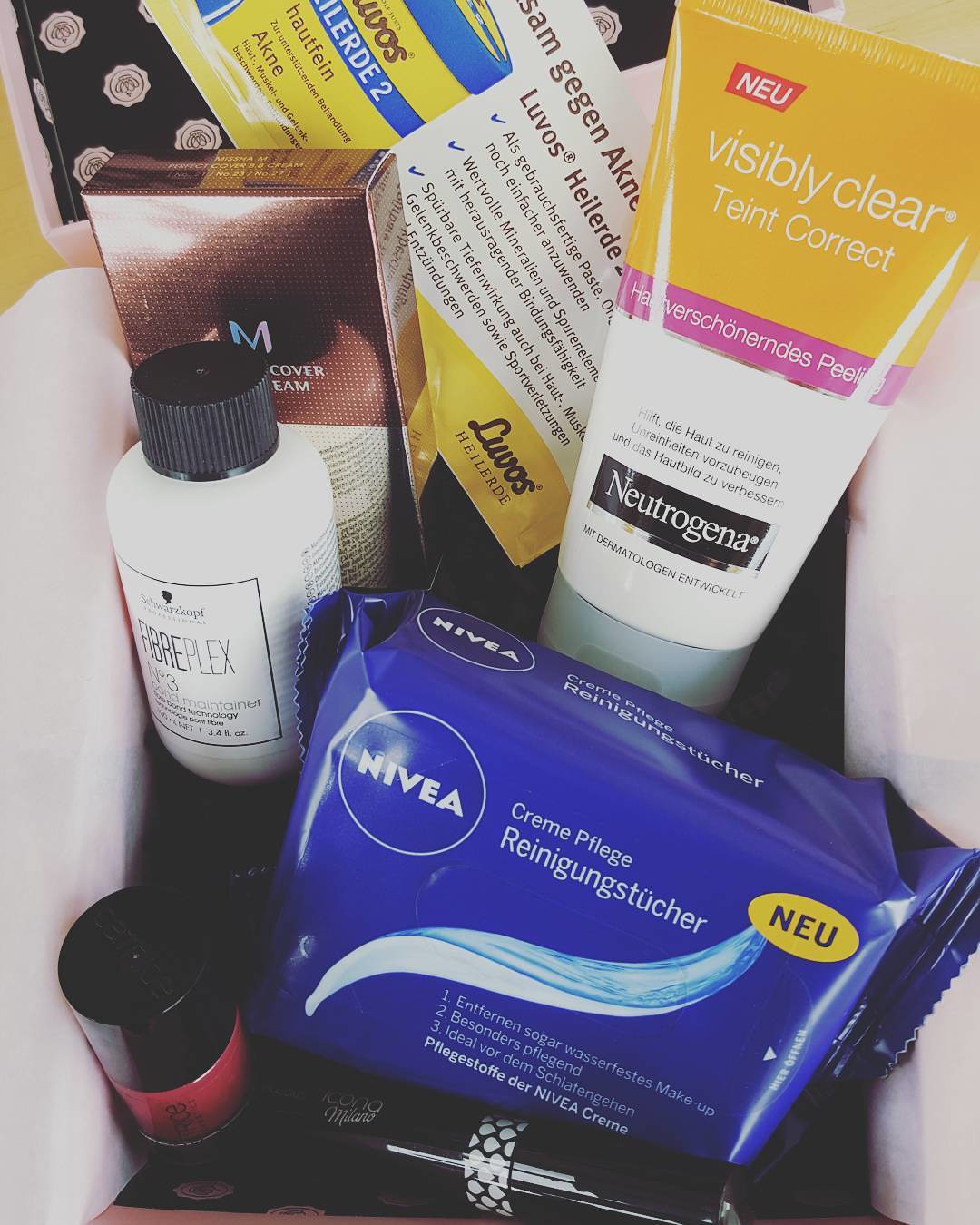This image appears to be an overhead view of a bathroom cabinet or drawer, organized into distinct sections or compartments. The sides of the enclosure are white, with a black bottom, contrasting vividly against the mosaic of personal care items strewn within. 

Starting from the lower left corner, there is a bottle of what seems to be a cosmetic product, possibly lipstick or lip gloss, characterized by a black cap and a red substance inside. Adjacent to it, a black tube decorated with a black and white honeycomb pattern lies on its side. 

Moving towards the center, a rectangular blue and white package of Nivea, possibly containing towelettes, labeled "Dren Schlegg Reine Gummstücke," hints at German origins. Extending from the upper right corner and spanning towards the center is a yellow and white tube of Neutrogena's "Visibly Clear" product, identifiable by a pink streak across its middle and white printed words.

In the immediate background, a yellow and white envelope with predominantly German text suggests additional facial care products or towelettes. The upper left corner houses a metallic, copper-colored tall box which likely contains more cosmetic items.

Finally, towards the middle left section, you can spot a small white bottle with plain black text and a matching black cap, completing this detailed glimpse into a meticulously stocked personal care collection.